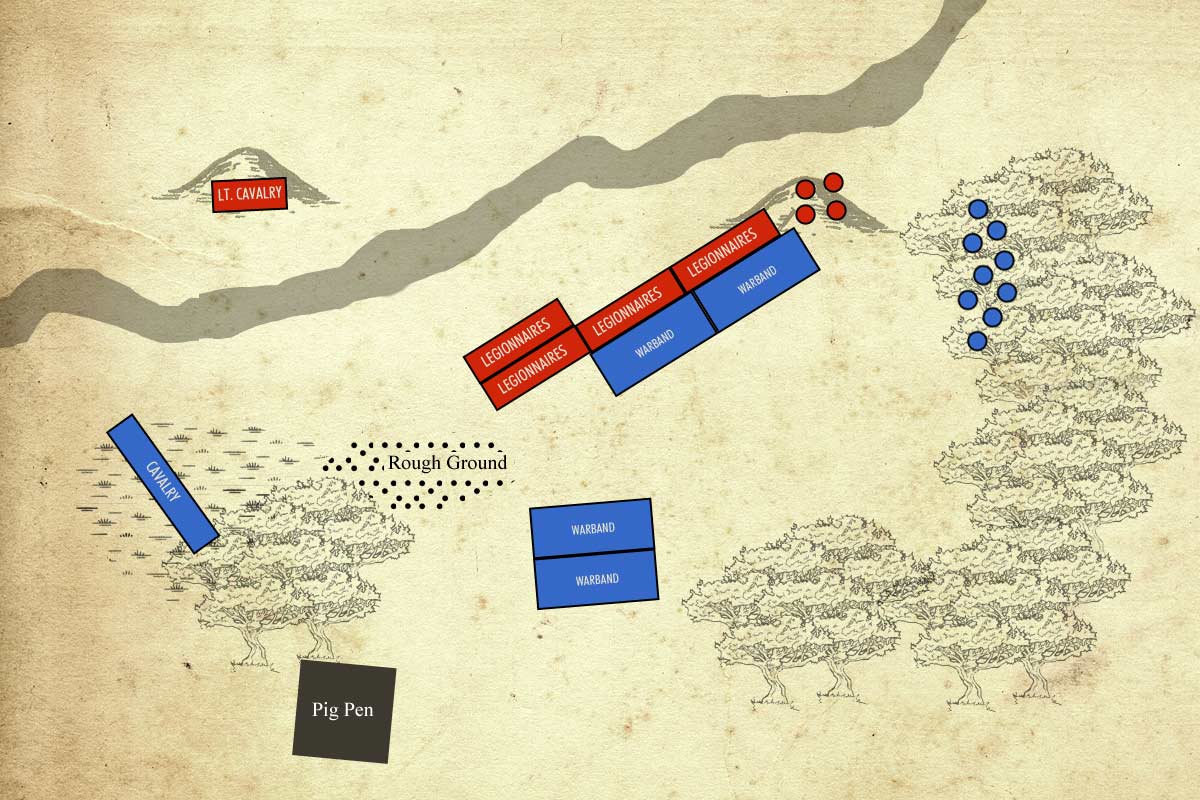The image depicts a detailed battlefield map, likely designed during a competition or wartime strategy session. In the upper left corner, on a gray mountain sketched with a red background, the label "L.T. Cavalry" stands prominently in white letters. A gray line, resembling a river, runs diagonally from the left center to the upper right corner of the map, effectively dividing the battlefield.

In the bottom left quadrant, a blue background with white letters prominently marks "Cavalry" beneath illustrations of trees. Adjacent to it, over a gray background with white text, is an area labeled "Pigpen." To the right of this section is another blue background with white lettering that reads "Warband," surrounded by sketches of trees extending upwards towards the center.

Centrally located are four red rectangles labeled "Legionnaires" in white letters. Below these, two blue rectangles also marked "Warband" lay opposite the four red boxes. Additional red dots, possibly representing units or key positions, are positioned near another mountain in the background, while eight to nine blue dots cluster in the right-center region, mingled within tree sketches.

The overall topography includes a significant knoll on the right side adorned with red and blue dots, indicating strategic positions. The map also identifies an area marked "rough ground," suggesting terrain considerations for the cavalry's movement. This intricately detailed map offers a comprehensive overview of the battlefield's layout, troop deployments, and significant natural features.